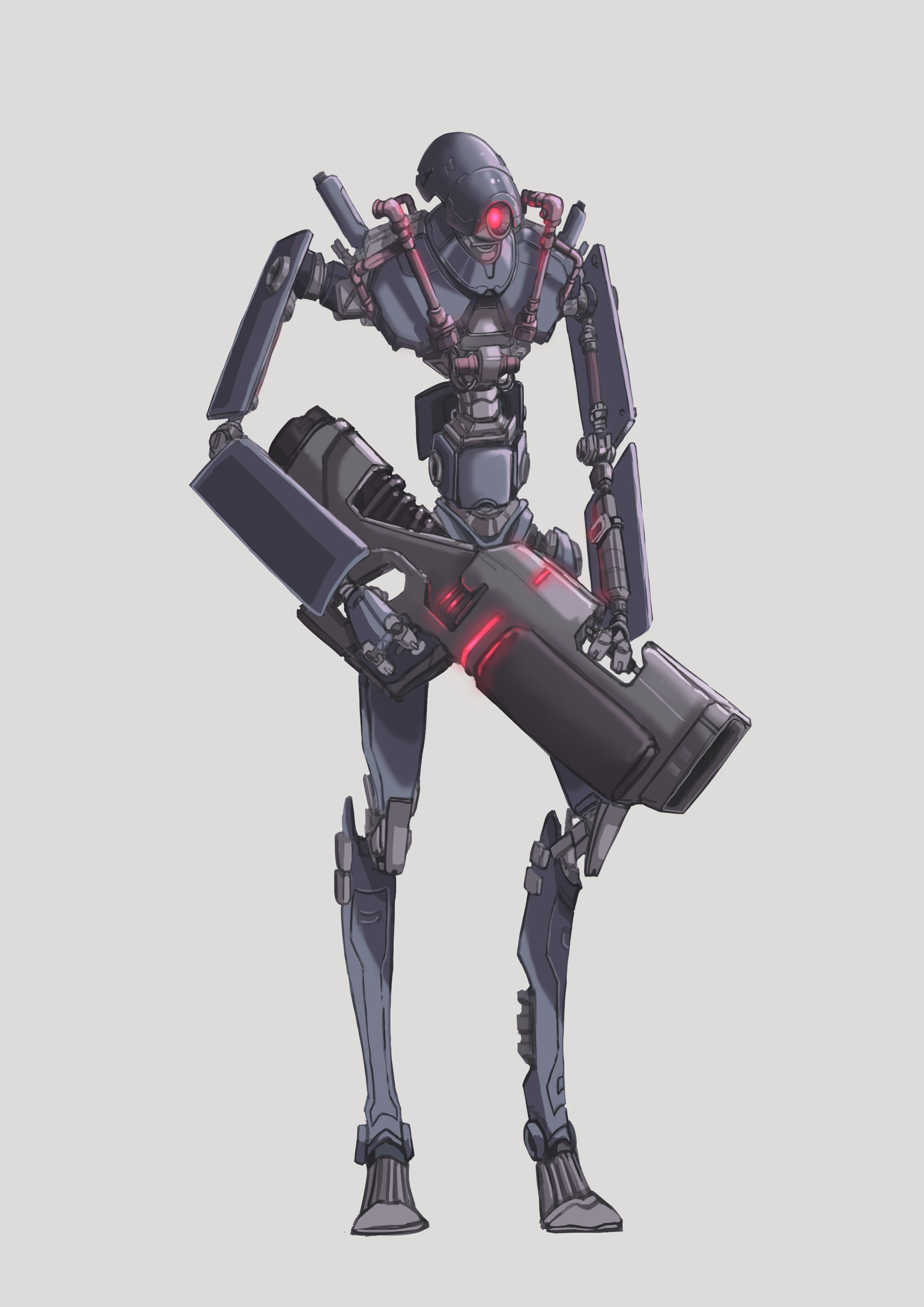The image is a vertical, computer-generated illustration set against a light beige background. It features a tall, slender robot with a humanoid form, characterized by thin limbs, a narrow torso, and a bug-like head. The robot is primarily gunmetal gray with intricate detailing that includes pipes, bolts, and hinges, giving it an alien-like, cybernetic appearance. A single, glowing red light in the center of its head serves as its eye, similar to a security camera. The robot grips a large, metallic gun with its right hand, which also features red lights, suggesting it could be a laser weapon. The scene shows the entire robot standing in a neutral pose, highlighting its structure and the detailed design of both the robot and its weapon. There is no text in the image.